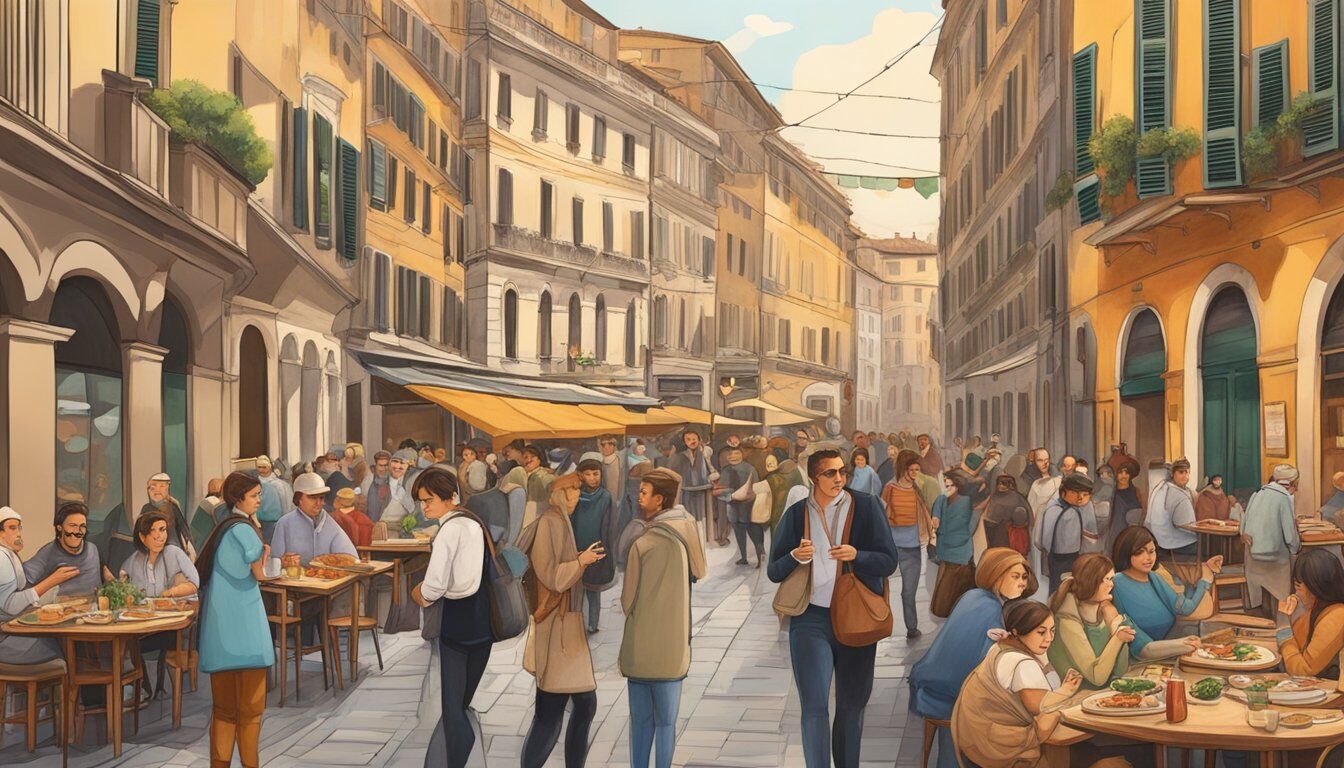The image is a rich, detailed painting of a bustling European street scene, which has a somewhat cartoonish, computer-generated feel to it. The narrow, cobblestone street is flanked by tall, tan and light yellow buildings, possibly four stories high, many of which feature shutters, and some have clotheslines displaying hanging garments alongside potted plants in the windows. The sky overhead is a vibrant blue with a smattering of clouds. The street, which might be better described as a courtyard or boardwalk area, is lined with numerous tables on both sides, where people are sitting, eating, and drinking, dressed mostly in casual attire with coats, hinting at cooler weather. The scene is alive with activity, as people walk down the middle of the street and gather in groups to talk, creating a sense of a busy, vibrant community. The overall ambiance and architectural style suggest this could be an urban setting in Italy.